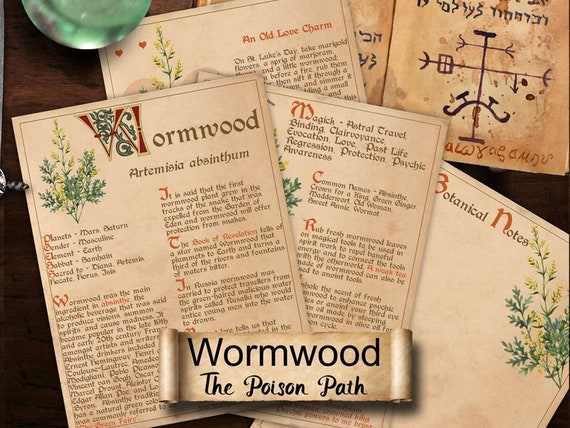The image depicts a collection of papers scattered across a brown table. In the foreground, there is a prominent depiction of an unrolled scroll or banner with black text that reads "Wormwood, The Poisoned Path" in large, bold lettering. This title appears multiple times across the various pages. These pages, mostly pink in color except for one that seems brownish, have intricate and detailed text, sometimes decorated with ornate, medieval-style fonts, especially on the page with "Wormwood, Artemisia Absinthe" written on it. Surrounding these central documents are additional papers containing various texts and possibly illustrations related to witchcraft, botanical notes, and an old love charm. One page even appears to have Hebrew writing accompanied by a diagram resembling an arrow or wind vane. In the upper left corner, there is a small glass or vase-like object, which might contain water, and a green sphere. The arrangement suggests a theme involving historical or mystical elements, particularly focusing on Wormwood and its uses or symbolism.